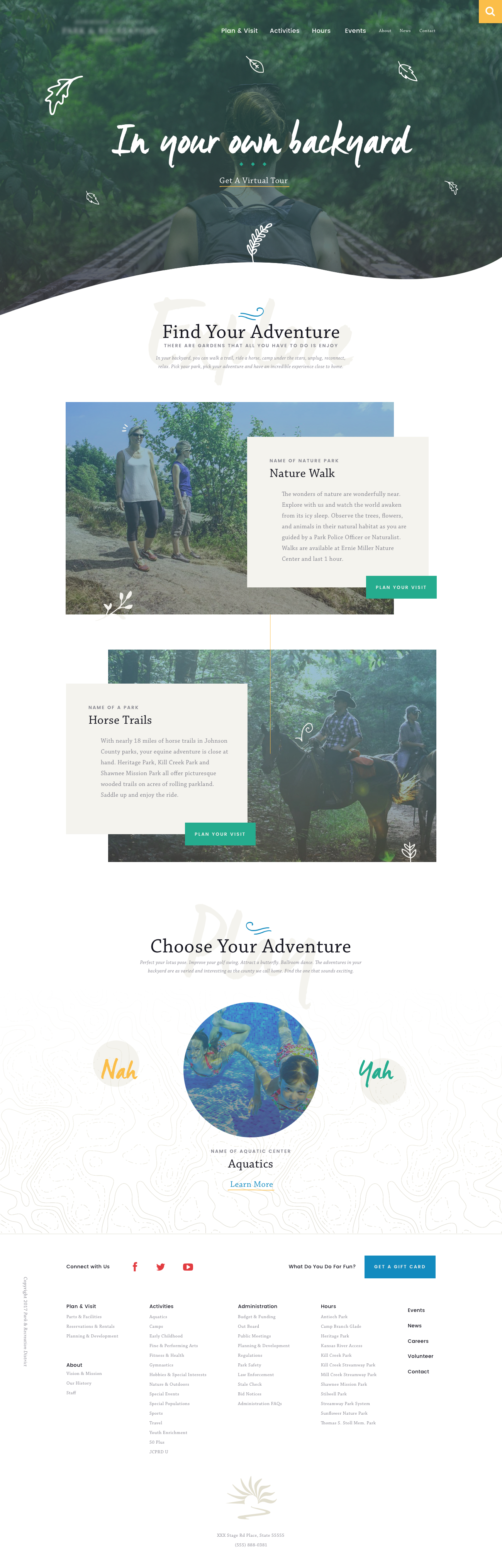The image features a lush, vibrant green banner that instantly captures attention with its depiction of verdant trees, rich grass, and dense foliage. The top portion of the banner includes a navigation bar with at least five clickable options for more detailed exploration. Prominently displayed across this green expanse is the phrase "In Your Backyard," written in a bold, stylized cursive font in white, accompanied by a falling leaf design, also in white.

Beneath this, the text "Find Your Adventure" stands out in bold black lettering, though the sentence that follows is rendered in such small font that it is difficult to read. Further down, an image depicts a couple walking along a picturesque pathway through the greenery, captioned "A nature walk," followed by another barely discernible paragraph.

The banner also highlights horse trails, showcasing people riding horses for those interested in equestrian activities. Finally, at the bottom, the caption "Choose Your Adventure" is displayed alongside a picture of the world, suggesting a variety of nature destinations available for exploration.